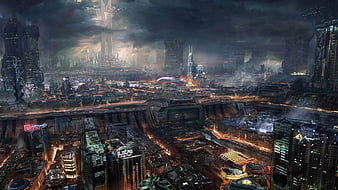The image is a small rectangular graphic, approximately two inches wide and one inch high, resembling a painting or a still shot from a movie. It vividly portrays a bustling cityscape, divided horizontally by what appears to be a large metal or stone dam-like structure. The lower half of the image showcases the city's lower levels, illuminated with vibrant orange, yellow, and blue lights, possibly indicating lively streets or buildings. Above the dam, the cityscape continues with towering skyscrapers reaching up towards a dark, cloud-laden sky, emphasizing a stark contrast between the bright city lights and the foreboding heavens. Just left of center at the top, a prominent light brown building stands out, glowing amidst the darker surroundings, suggesting a source of illumination or significance within the urban landscape. This intricate and colorful depiction, which could be a scene from a video game, captures a dynamic and vibrant urban environment.